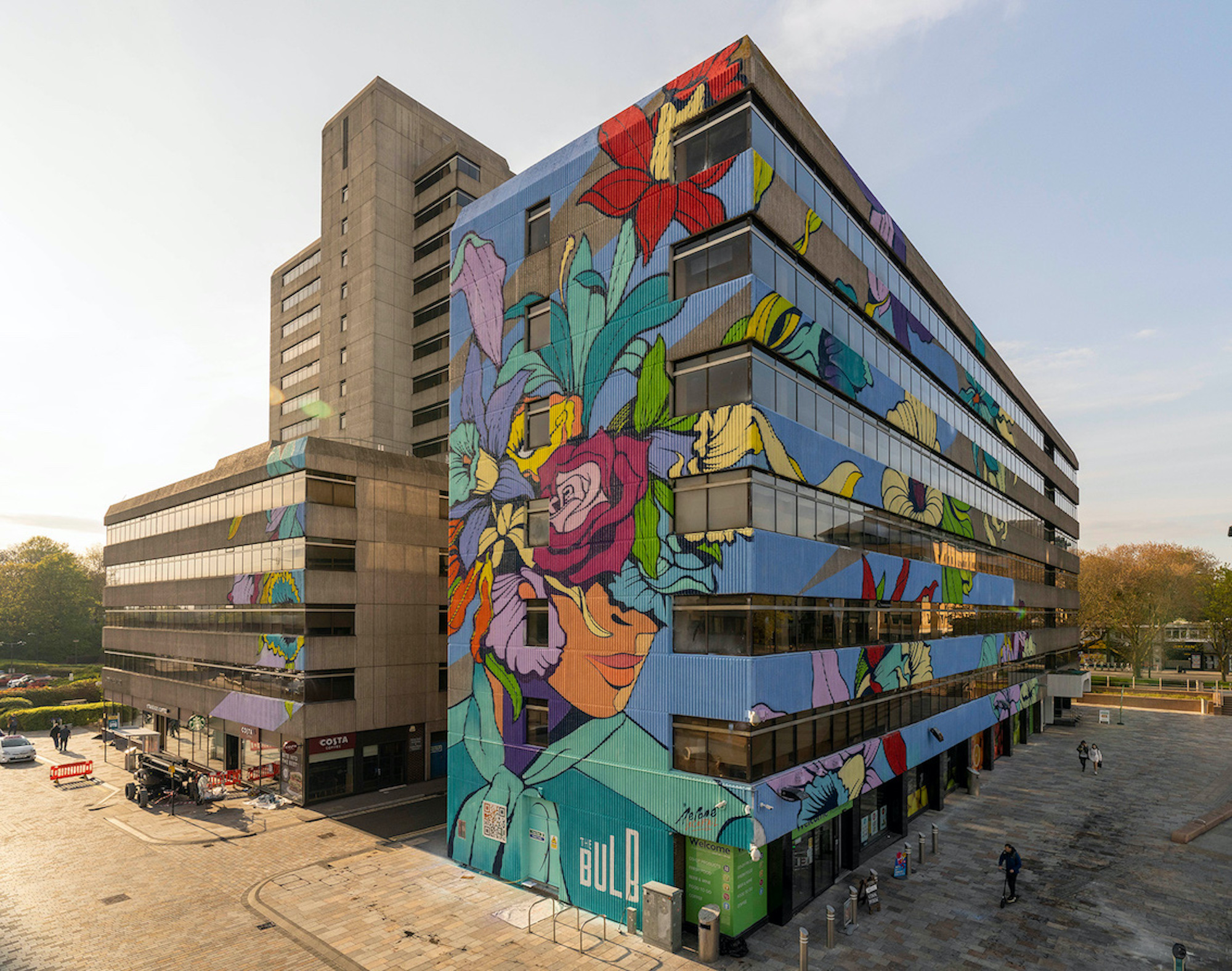The photograph captures the exterior of two distinct buildings from an angled perspective, with the camera positioned near the right-hand corner of the building on the right. The focal point is a seven-story, rectangular building on the right, adorned with an expansive mural covering its shorter side. This mural features the vibrant image of a Black woman with flowers emanating from her head and a turquoise scarf around her neck, set against a blue background. The building's continuous strips of windows on each story are visible through the artwork, giving it a dynamic visual appeal. 

To the left, there stands a larger, more industrial-looking structure made predominantly of gray concrete blocks. This building has a base of five stories, with an additional narrower tower reaching up eight more stories. Its façade is simple, with a series of black windows on the lower floors. The area in front of this building is characterized by wide sidewalks, a street with a car park, and minimal vegetation, suggesting a new development. There is a genie lift machine at the base, hinting at recent or ongoing construction activities. The entire scene is set against a bright blue sky, with some smaller trees in the background, providing a stark contrast to the urban landscape.